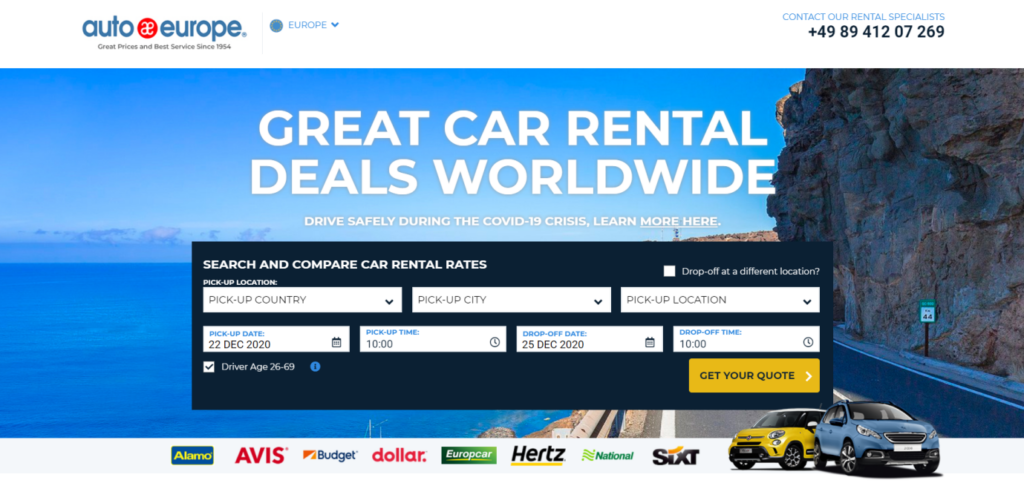Screenshot of the Auto Europe website. The homepage prominently features the tagline "Great Car Rental Deals Worldwide" in bold white text. The background image depicts a breathtaking coastal scene with a vast ocean to the right, a rugged cliff face to the left, and a clear, expansive sky above. The interface includes dialogue boxes at the top for users to input rental details. At the bottom, logos of various car rental companies such as Avis, Budget, Dollar, and Hertz are displayed alongside images of cars. The website serves as a comprehensive aggregator for car rental services. A customer service phone number is also visible, ensuring users can easily reach out for assistance.